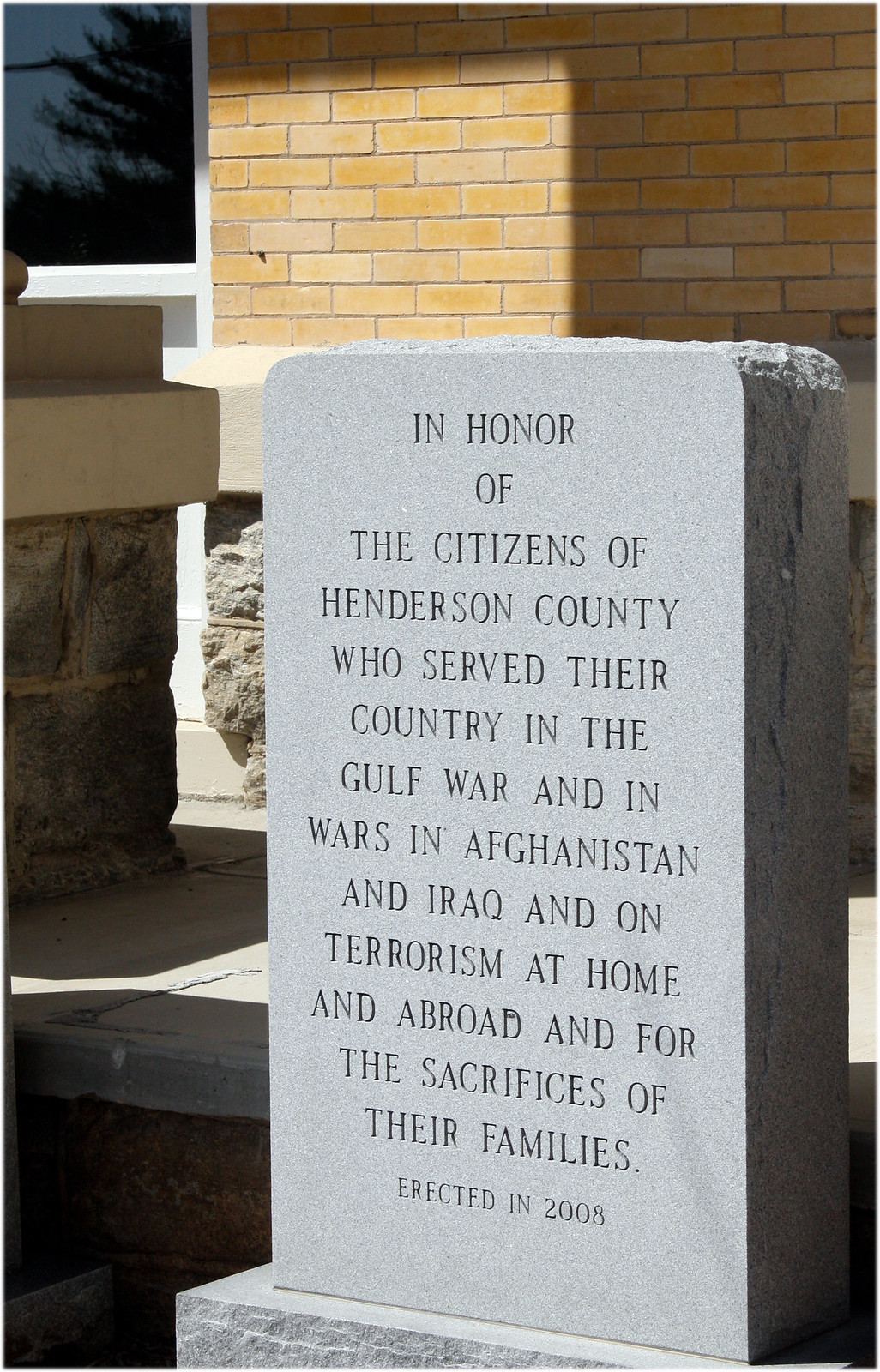The image captures a gray stone memorial resembling a grave marker, resting on a platform with notable features such as a polished face and rugged top. The inscription on the memorial reads: "In honor of the citizens of Henderson County who served their country in the Gulf War and in wars in Afghanistan and Iraq and on terrorism at home and abroad and for the sacrifices of their families. Erected in 2008." The text is carved in capital letters. Positioned to the right side of the memorial, some cracking is evident. Behind the memorial stands a building characterized by a brick wall with stone trim at the bottom and a window partially visible, adorned with black frames and white borders. The photograph is taken during daylight, with sunlight illuminating the wall, floor, and memorial, enhancing the contrast of the gray, tan, black, and white colors in the scene.